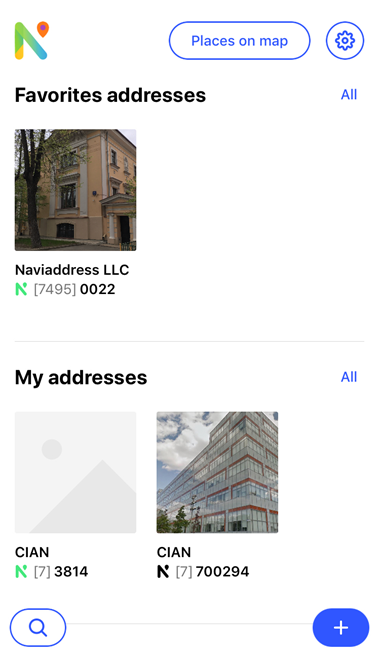This image is a screenshot from the Google Maps app, showcasing a predominantly white background. In the top left corner, there's an icon depicting a green, yellow, and blue inverted V-shape, adjacent to an orange teardrop symbol with a purple interior. To its right, the phrase "Places on Map" is displayed within a blue oval. A settings icon, represented by a circle encompassing a cogwheel, is positioned nearby.

Below this, the interface reads "Favorite Addresses" followed by "All." There is a thumbnail image marked "Nav Address LLC, [7495] 0022" in bold. Further down, "My Addresses" is prominently displayed in dark black with "All" highlighted in blue next to it. 

The next section includes two boxes. The first box is a placeholder image labeled "Cyan [7] 3814." The second box contains an image of a tall building, surrounded by trees, a blue sky, and white fluffy clouds, labeled "Cyan [7] 700294."

At the bottom of the screenshot, a blue search bar and a blue plus sign are visible, likely offering additional functionalities within the app.